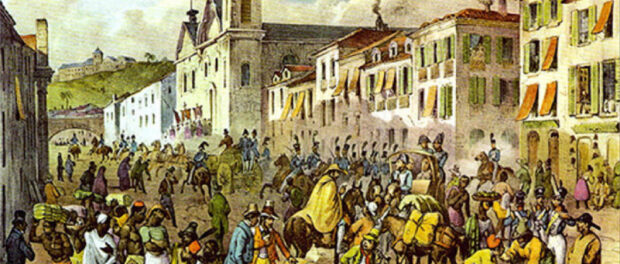An old-fashioned painting captures a bustling city street from a bygone era, where horses and horse-drawn vehicles dominate the scene. The focal point features several figures on horseback dressed in blue uniforms and tall hats, suggesting they might be law enforcement or colonial officers. These figures are depicted with minimal detail, giving a sense of movement and busyness. 

In the foreground, locals dressed in casual attire, some even shirtless, populate the scene, indicating a warm climate. The crowd presents a vivid contrast with the more formally dressed individuals on horseback, highlighting the diverse social dynamics at play. 

To the right, a row of tall buildings, possibly homes or apartments, lines the street, while the path underfoot is unpaved, hinting at the simplicity and rustic nature of the setting. In the background, a gentle green hill rises, providing a serene counterpoint to the lively street below. The dirt road is busy with people going about their day, creating a lively and dynamic atmosphere.